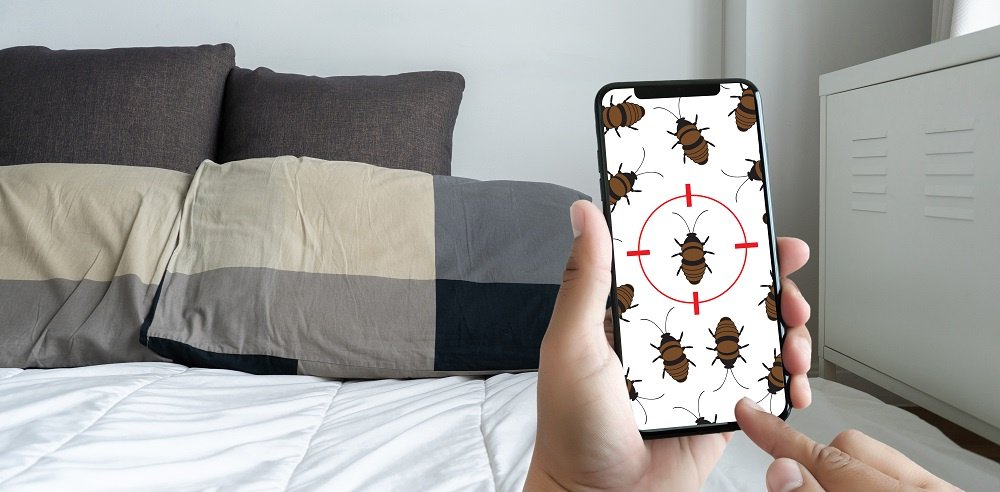The photograph is an indoor scene, horizontally rectangular in shape, showcasing a cozy bedroom setting. Dominating much of the image is a neatly made bed with a white comforter, topped with several pillows in various shades: dark brown ones in the back, followed by mixed hues of cream, gray, light gray, and black, including some with a checkered pattern. To the right, a modern white cabinet with vent-like slats is partially visible. The backdrop includes pristine white walls.

In the lower right-hand corner, a pair of Caucasian hands are holding an iPhone. The left hand grasps the phone while the right hand appears ready to interact with the screen. The phone's display shows a white background populated by brown and black cockroaches, with a red crosshair target positioned over the centermost cockroach, suggesting that the user is engaging in a game aimed at exterminating the insects. The absence of nail polish on the fingers and the presence of natural lighting complete the detailed composition.